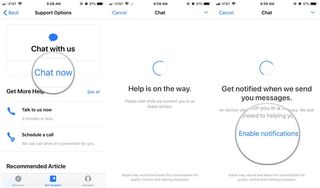The image is a composite of three vertically aligned screenshots taken from an iPhone, forming a long rectangular shape. Each screenshot appears slightly blurry with a white background, likely representing a sequence of steps for engaging with Apple Support. 

In the first screenshot, a section titled "Support Options" is visible on the left side. It features a blue speech bubble icon accompanied by the text "Chat with us" in black, indicating the option to initiate a live chat with Apple Support. Below this, a clickable "Chat now" button is highlighted by a grey circle superimposed over it, directing users to start the chat.

The middle screenshot shows the next step in the process, displayed as a moving circle, suggesting a loading or processing state. The text "Help is on the way" appears in black, with some unreadable grey text beneath it, likely providing additional context or information.

The third and final screenshot continues with the loading circle motif. Below it, a message reads "Get notified when we send you messages," followed by an "Enable notifications" option in blue text. This option is also emphasized by a superimposed grey circle, highlighting the importance of enabling notifications for ongoing support updates.